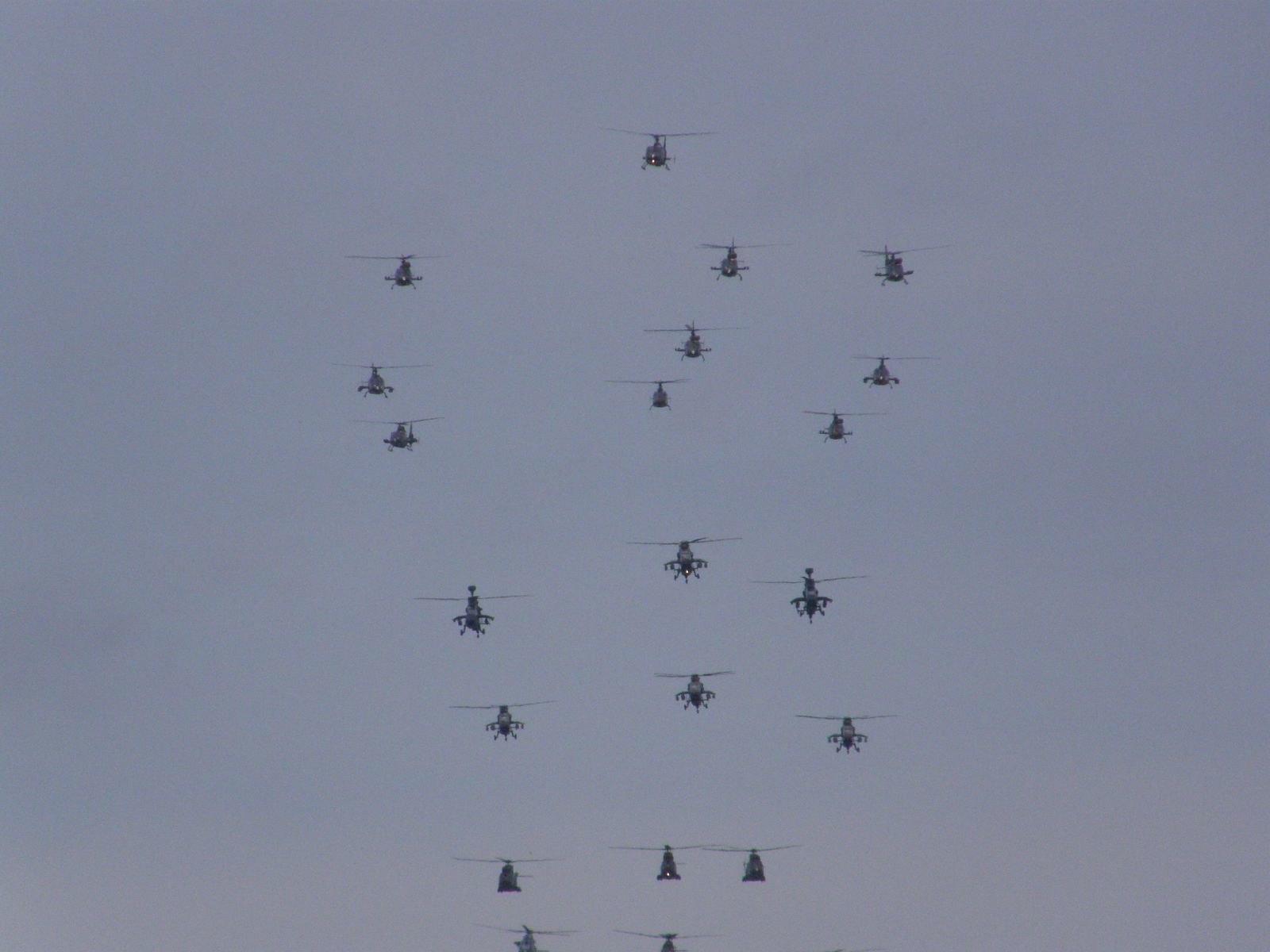This photograph captures an impressive aerial formation of 21 military-style helicopters flying toward the camera, set against a predominantly gray, overcast sky. Dominating the center of the image are multiple gunships, each equipped with visible pods, likely housing rockets. At the top of the formation, we observe Huey-type helicopters reminiscent of the Vietnam War era, featuring rounded fronts. Positioned below them are smaller, four-bladed medical-style helicopters with faster-spinning rotors. The lower section of the image showcases heavier helicopters, possibly with amphibious landing pontoons on their sides, further emphasizing their formidable presence. The formation is organized into one helicopter leading, followed by three distinct rows of three, another group of six in a less structured arrangement, succeeded by two more rows of three, another row of three, and finally a concluding pair of helicopters. While the hue of the sky conveys a possible cloudy day, the meticulous arrangement and varying designs of the helicopters create a striking and detailed tableau.